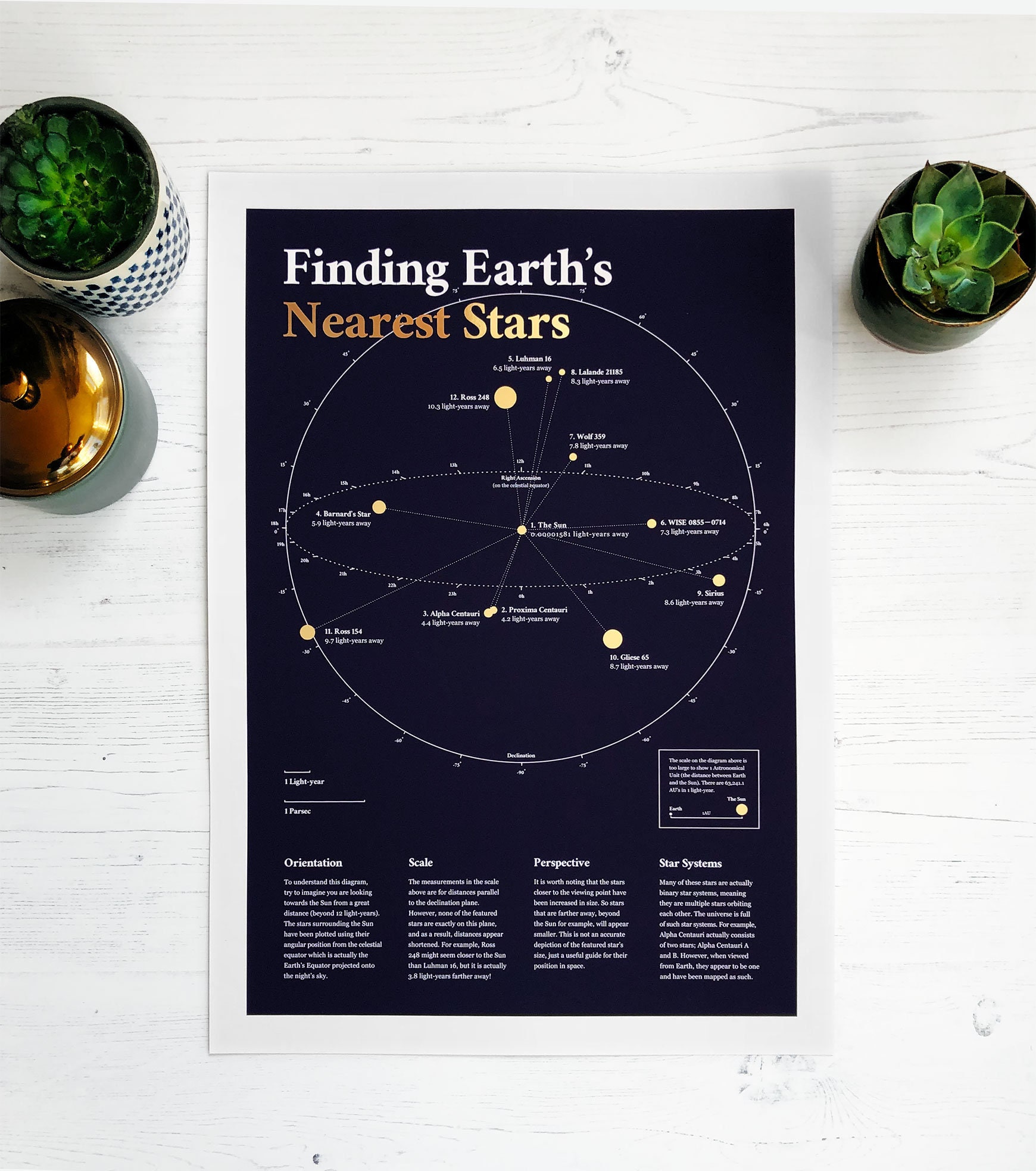A magazine page or a poster, approximately five inches high by four inches wide, lays flat on a whitewashed wooden tabletop. Flanking the poster are two succulent plants; one in a square white and blue pot and another in a can, with a little container featuring a copper lid situated near them. The poster itself is rectangular with a light grayish-white border and features a deep navy blue background. In white text at the top left corner, it reads "Finding Earth's Nearest Stars," with "Nearest" highlighted in orange and "Stars" in yellow. A large white circle dominates the center of the poster, depicting the orbits of celestial bodies, including planets and stars, arranged in concentric circles with arrows indicating their positions. The poster further breaks down its information into four paragraphs at the bottom, labeled from left to right: Orientation, Scale, Perspective, and Star Systems.